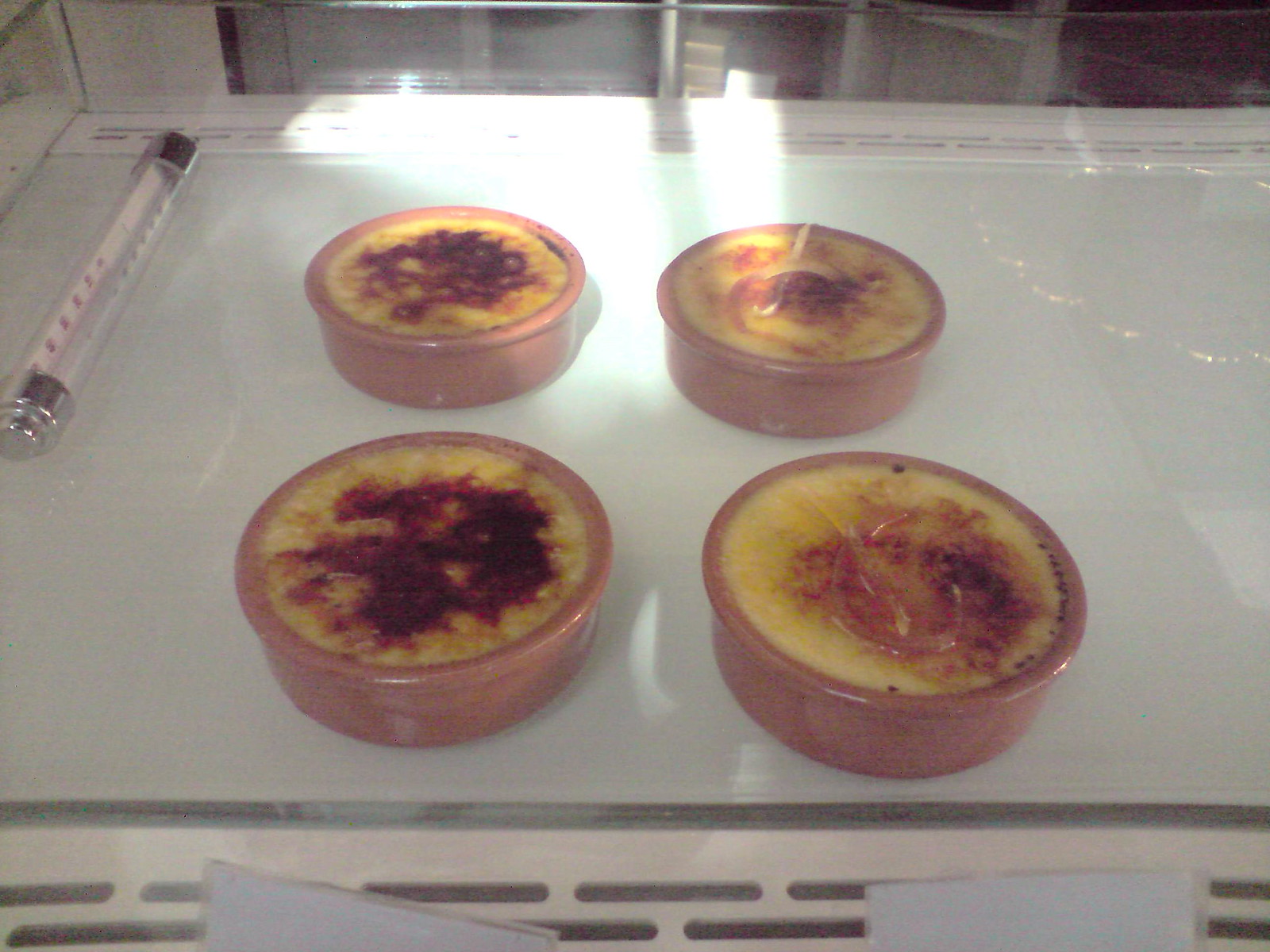The photograph captures four creme brulee desserts arranged in a square formation in dark pink, earthenware ramekins on a white appliance surface, likely within a commercial kitchen. The viewing angle is slightly downward, revealing an industrial thermometer resting on the top left of the image. Sunlight gently illuminates the two ramekins on the right. Each creme brulee displays a varying degree of caramelization, with the dessert in the front left showing the most scorching. Behind the desserts, blurred shelves are faintly visible, reinforcing the bustling kitchen environment.